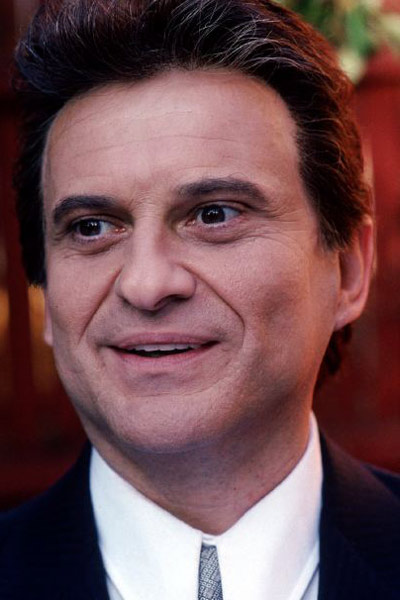The photograph captures what appears to be Joe Pesci, the renowned Italian-American actor known for his role in "My Cousin Vinny." The image seems to date back to the 1980s, showcasing him from the neck up in a tall rectangular format. Pesci, a Caucasian man with a slightly amused and good-natured expression, has short, thick, dark brown hair styled in a low bouffant manner, with a hint of gray along his hairline. His eyes, glowing with a respectful gaze, are directed slightly to the left. He is clean-shaven, his brown eyebrows accentuating his brown eyes. Pesci's mouth is slightly open, revealing the top of his teeth as he smiles gently.

He is dressed in a classic ensemble of a white collared shirt fully buttoned up and a finely striped tie with diagonal blue and white stripes. Completing his attire is a black suit jacket, though only part of it is visible within the frame. The background consists of a light orangey-brown hue, with a notable green spot in the upper right corner. Additional elements behind him include what appears to be pieces of wooden furniture and potentially the front and back of a car, hinted at by red and mostly vertical lines, and a mix of colors and shapes that blend into a slightly blurry form in the background.